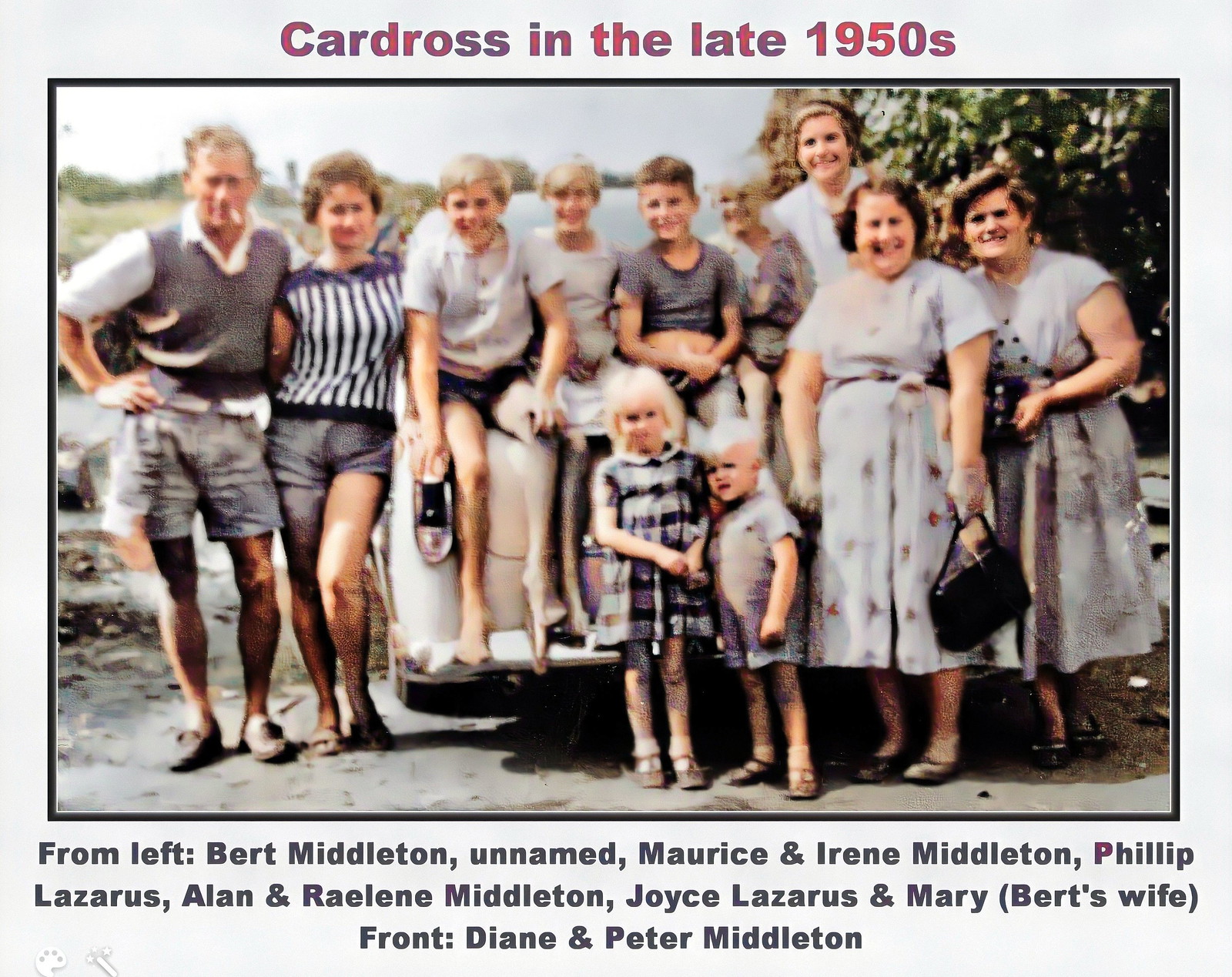The image is a wide, rectangular, framed photograph with a light blue border. At the center is an old-fashioned photograph captioned at the top in purple and pink font: "Carr-Dross in the late 1950s." The bottom of the frame reads in dark gray font: "From left: Burt Middleton, unnamed, Maurice and Irene Middleton, Philip Lazarus, Alan and Raylene Middleton, Joyce Lazarus and Mary (Burt's wife). Front: Diane and Peter Middleton." The photograph depicts a large group of people posing outdoors in front of a white car. Several individuals are seated on the car's hood, while others stand around it. In the front row, there are two young children with bright blonde hair. A man with blond hair, possibly holding a cigarette, stands to the left, with his arm around a woman in a white-striped shirt and shorts. To the right, elderly and middle-aged women, one holding a pocketbook, are positioned beside the children. The background features green grass and trees, indicating an outdoor setting.